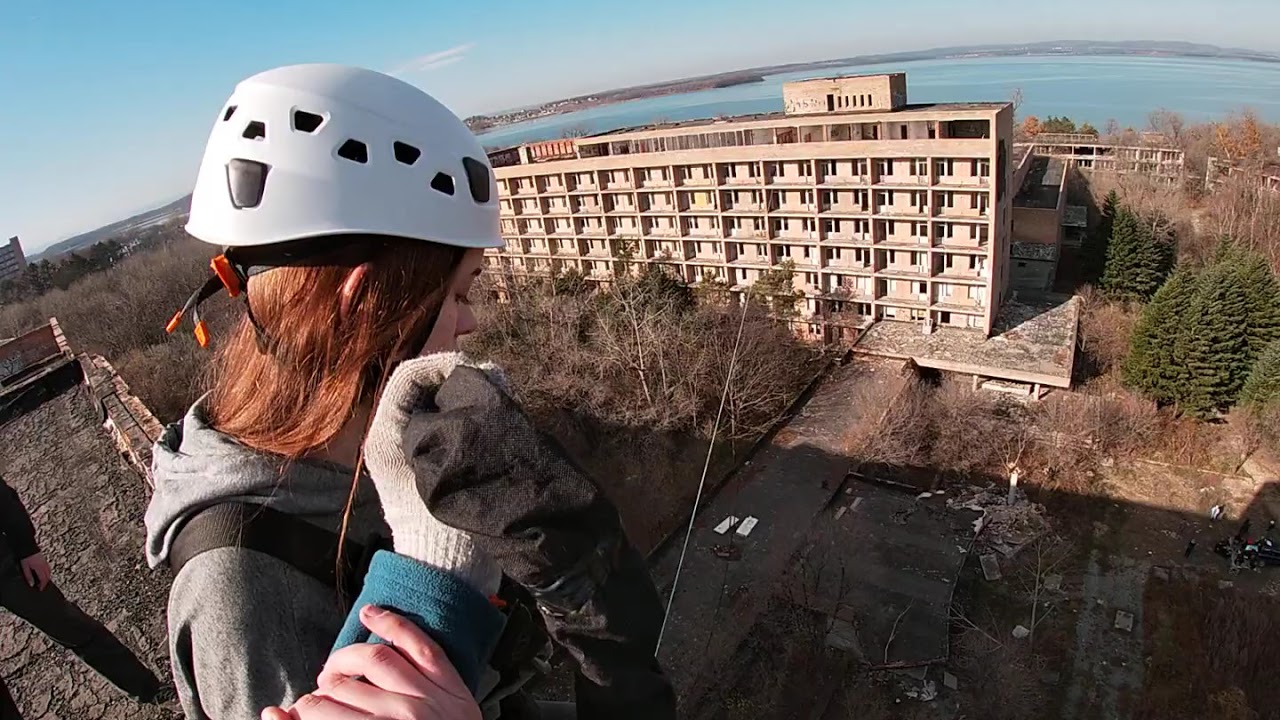From a high vantage point on a rooftop, the photo captures a detailed outdoor scene under a sunny, clear blue sky. In the background, a body of water that appears to be a lake stretches to a distant, brown shoreline. Dominating the right side of the frame is a large, multi-story building that could be an apartment or hotel high-rise. At ground level below, a patch of brown dirt is visible, along with scattered remnants suggesting a demolished building. Sparse, leafless trees add to the stark landscape, save for a few green pine trees providing a hint of color. 

On the rooftop, a woman with reddish-brown hair is seen wearing a white helmet, a gray hoodie, and gloves. She appears to be carefully positioned near a zip line strung between two buildings. The woman seems to be holding someone's hand, likely for balance, as they wear a teal jacket and light gray gloves. Additionally, another individual dressed in black is spotted further to the left on the rooftop. The image conveys a mix of urban decay and human presence, highlighted by the contrasting greenery and expansive blue skies.